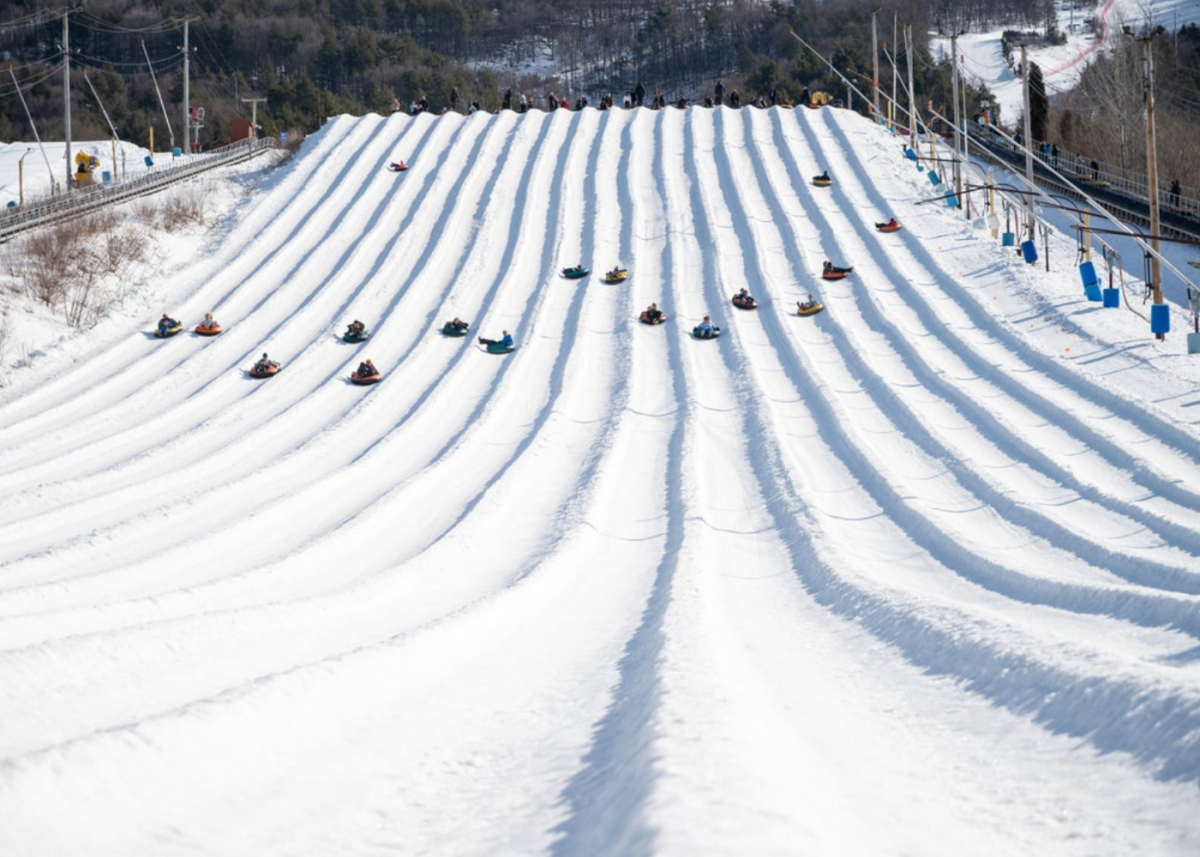This photograph captures a bustling snowy tubing hill from a bottom-up perspective. The scene features approximately 17 distinct tubing lanes, each separate by raised snow walls that act like railings. At the top of the hill, a crowd of people is visible, eagerly waiting for their turn. Down in the lanes, around 15 tubers are in mid-descent, some riding solo while others share their tubes, with a few even sliding backwards. The hill is flanked by various details: poles with blue cushions on the right, a fence on the far left, and what appears to be a walkway or tramway running up the hill's left side, likely for climbers. The background is lined with snow-covered trees on additional hills, all enveloped in a chilly winter atmosphere. The tubers appear small and slightly blurred, emphasizing the grandeur and activity of the snowy hill.